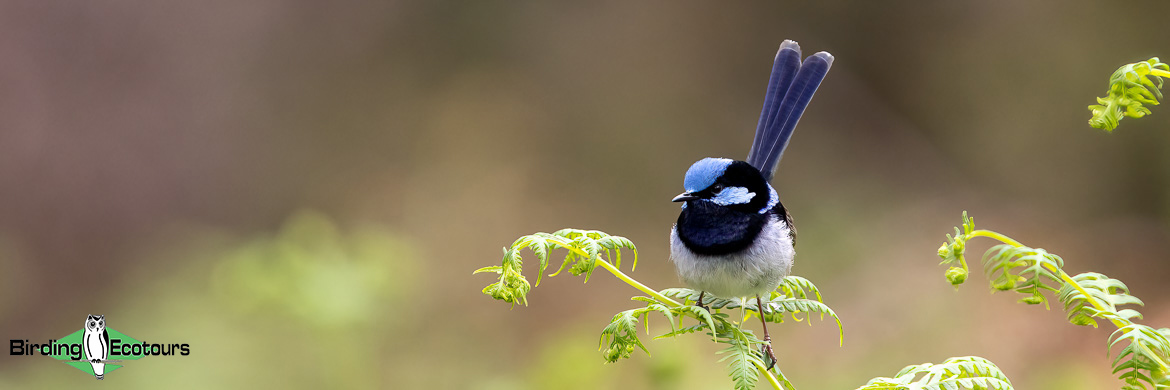This high-definition photo captures a small, round bird with distinctive markings. The bird's head features a light blue forehead with black surrounding its eyes and extending toward the back of its head, which is accented by a black beak and black eyes. Its cheeks and underbelly are white, while the throat area is marked by a band of black that extends down the front of its body. The bird's back is also white, complemented by its dark brown stick-like legs. Two long, navy blue tail feathers with white tips are visible, pointing upwards to the right.

Perched delicately on a thin green stem of a leafy plant, the bird is the focal point of the image, with additional green stems and leaves situated to its right. The background is artistically blurred, blending green and brown hues to highlight the subject. A logo on the bottom left corner of the image reads "Birding Encounters," featuring an owl illustration within a green diamond.